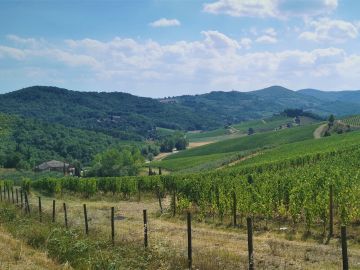In this captivating photograph of a picturesque countryside, the scene opens with a meandering dirt road that threads through the foreground, flanked by an old wire fence with sturdy posts stretching from east to west. The road meanders through a farmer’s field, lush with green vegetation that could be stalks of corn or another crop, though the exact type is indiscernible from the distance. Further back, rows of verdant trees populate the mid-ground, and beyond them, rolling hills gradually rise into a range of mid-high mountains. The mountains exhibit a deep green hue that transitions to a more turquoise shade as they fade into the distance. On the left side of the image, partially obscured by dense foliage, sits a modest house or structure. The house is nestled amongst the greenery, adding a quaint touch to the overall scene. Above, the sky is a light blue expanse, adorned with puffy white clouds extending across the horizon. The combination of natural elements and man-made structures encapsulates the serene beauty of this idyllic rural landscape.